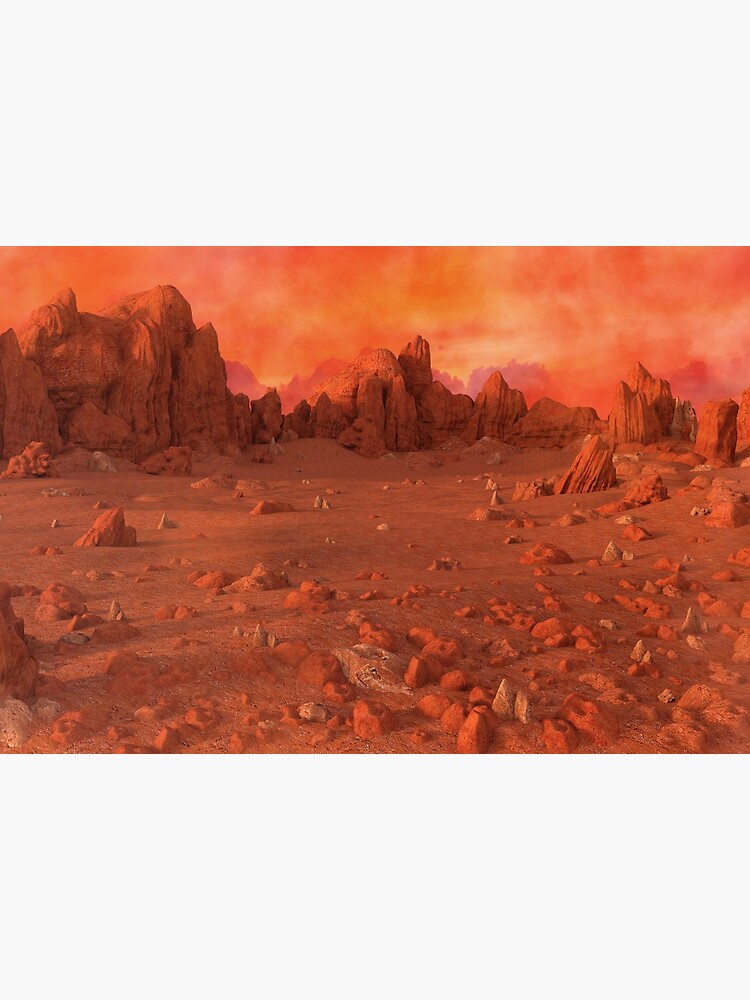The image portrays a stunning, fantasy-inspired landscape that resembles an extraterrestrial planet or a desolate wasteland. The scene is dominated by a rich palette of orange, gold, red, and hints of pink and gray. The jagged, rocky ground is strewn with sharp stones and slightly deeper red rocks that cast hazy shadows, creating a strikingly barren and otherworldly atmosphere. The horizon is marked by an array of cliffs and rock formations of varying heights and widths, starting from the tallest peaks on the upper left and gradually dipping and rising before tapering off to the right. The sky above is a mesmerizing swirl of bright oranges, yellows, reds, and pinks, reminiscent of a watercolor painting. The overall image is both a beautiful and stark depiction of a barren landscape, full of otherworldly charm and intrigue.